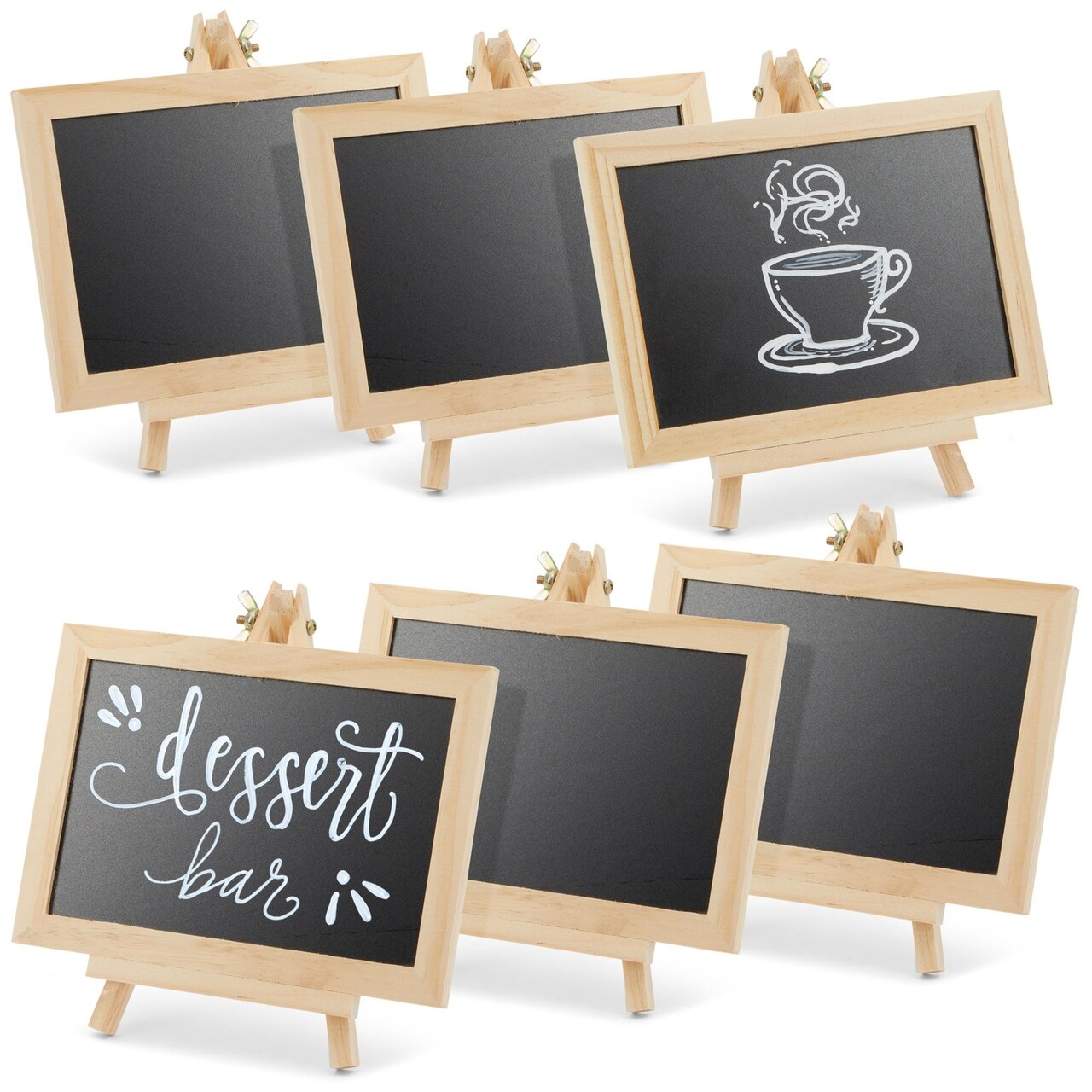The image displays six small chalkboards against a solid white background, arranged in two staggered rows. The top row consists of three chalkboards aligned diagonally from upper left to lower right, while the bottom row features three chalkboards aligned diagonally from lower left to upper right, creating a criss-cross pattern. Each chalkboard has a light-colored wood frame and small legs, resembling miniature easels.

The first chalkboard in the top row, positioned at the upper right, displays a white chalk drawing of a coffee cup placed on a saucer, with steam curling upwards elegantly. The corresponding first chalkboard in the bottom row, positioned at the lower left, features the words "dessert bar" written in white cursive script, along with a decorative design.

The overall arrangement and design are clear, with the overlapping positioning adding depth. The simplicity of the light wood frames and the blank chalkboards, aside from the highlighted designs on the front ones, makes each element easily distinguishable and visually appealing.